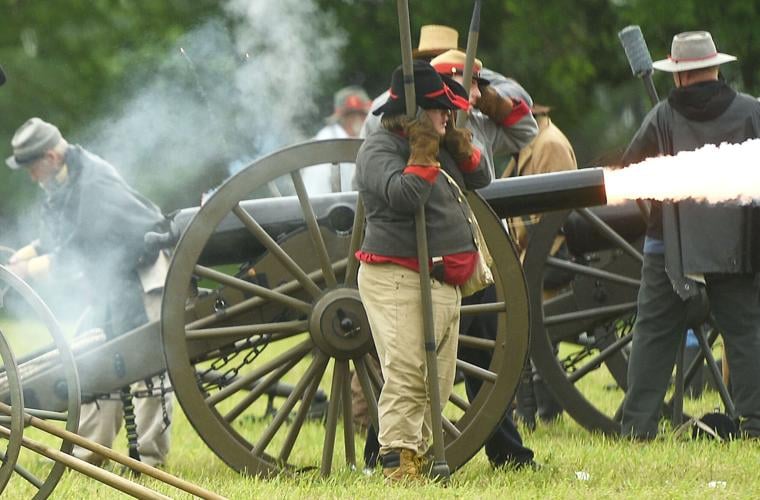In this detailed color photograph, a Civil War reenactment scene is vividly captured in a grassy field with darker green trees in the background. Central to the image is a large black cannon mounted on green wooden wheels and chassis, pointing to the right and emitting white smoke and flame as it fires. In the foreground stands a man dressed in a Civil War-era ensemble comprising a broad-brimmed black hat, a gray coat with red accents, tan pants, and leather gloves, though he is notably wearing modern boots. With a pike in hand and his fingers over his ears to muffle the cannon's roar, his tense posture implies the cannon has just fired. Behind him, a Union soldier dressed in a blue-gray uniform with a visor cap, along with other reenactors in period clothing and broad-brimmed hats, can be seen preparing additional cannons. These collective elements vividly depict the intensity and atmosphere of a historical battlefield.